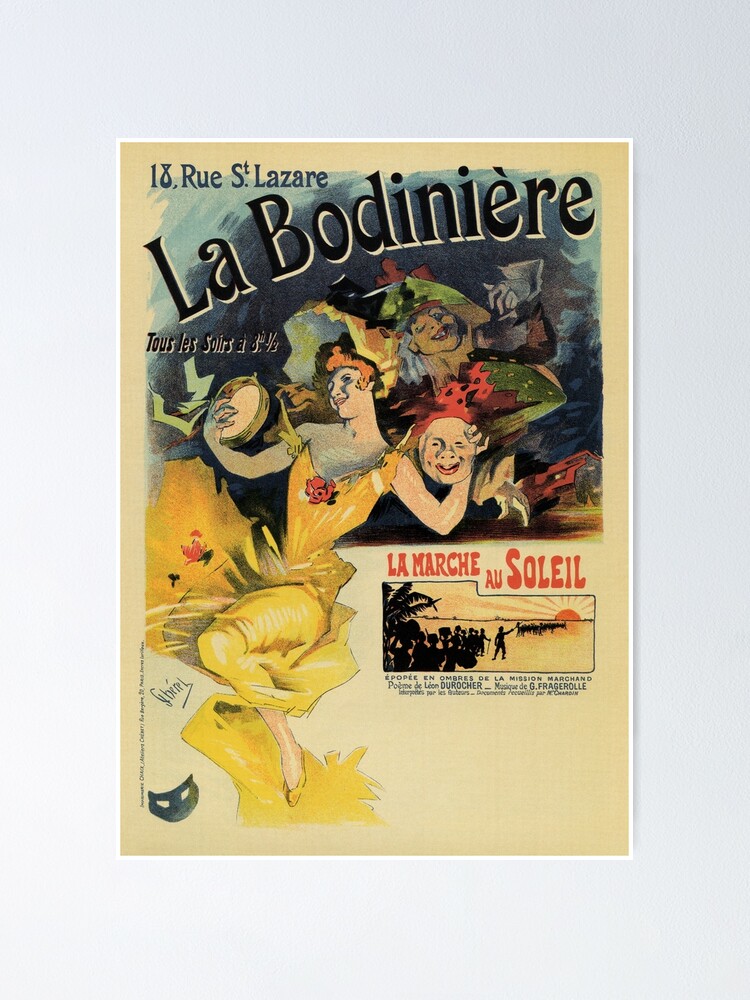This image, appearing to be an early 1900s magazine cover or a circus advertisement, features a striking, detailed illustration. The artwork, rendered in a cartoony, colored pencil style, predominantly displays a woman in a flowing yellow dress adorned with a red rose on her chest. She holds a tambourine in her right hand and a mask of a man in her left. She stands against a white background with peculiar characters in the backdrop, including distorted faces with pig-like features. The top right corner of the image shows a bluish-turquoise pattern, which includes the woman's face again. Beneath this is the red-text title, “La Marche au Soleil,” followed by a small landscape drawing of a sunrise or sunset with plants. The image is further marked by text including "La Boudiniere," “18 rue Saint-Laurice,” and other French phrases, indicating its origin and adding to its historic and adult-themed allure.